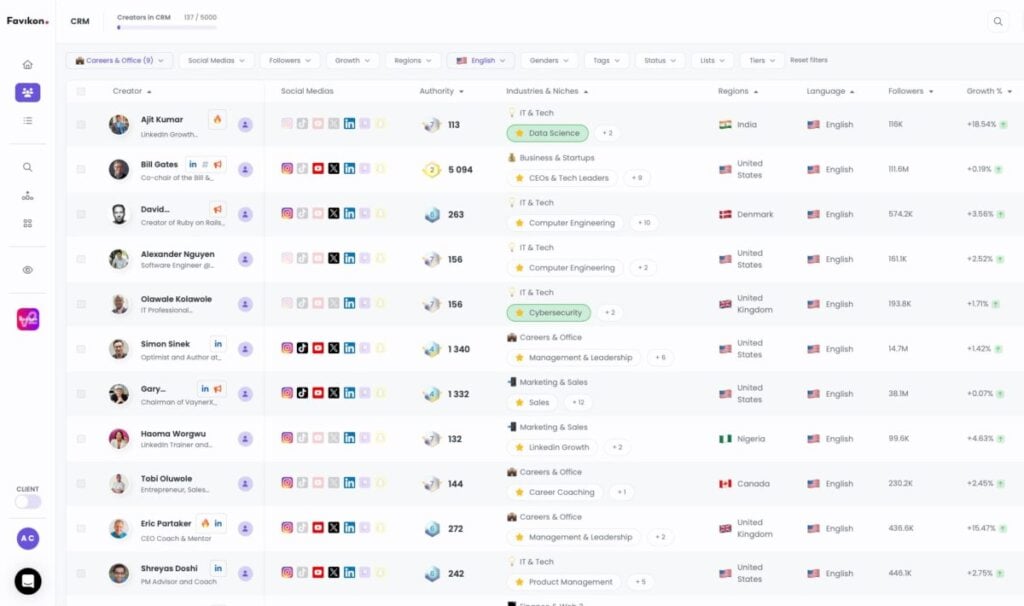The image appears to be a detailed screenshot of a web page that aggregates various social media profiles. The layout features a sidebar on the left, listing numerous individuals with a brief description of their professional roles, such as "LinkedIn Growth Coach," "Co-Chair," "Creator," or "Software Engineer." 

Alongside some of these profiles, there is a fire emoji, indicating perhaps trending or highly influential accounts. 

Each profile also includes icons representing the person's social media platforms, such as YouTube, X (formerly Twitter), LinkedIn, TikTok, and Instagram. 

Adjacent to the social media icons, there's a section labeled "Authority," which displays a numerical value, sometimes accompanied by a gold or silver icon, signifying their level of influence or credibility. 

Further details include the individual's industry and niches, for example, "IT and Tech," "Data Science," "Business and Startups," and "CEOs and Tech Leaders." 

The profiles also specify the individuals’ region, such as "India," "United States," or "Denmark," and the languages they speak, predominantly "English."

Lastly, follower counts and growth percentages are presented, providing insights into their social media growth dynamics. This web page seems to serve as a platform for tracking and showcasing the growth and influence of various professionals across different regions and industries.